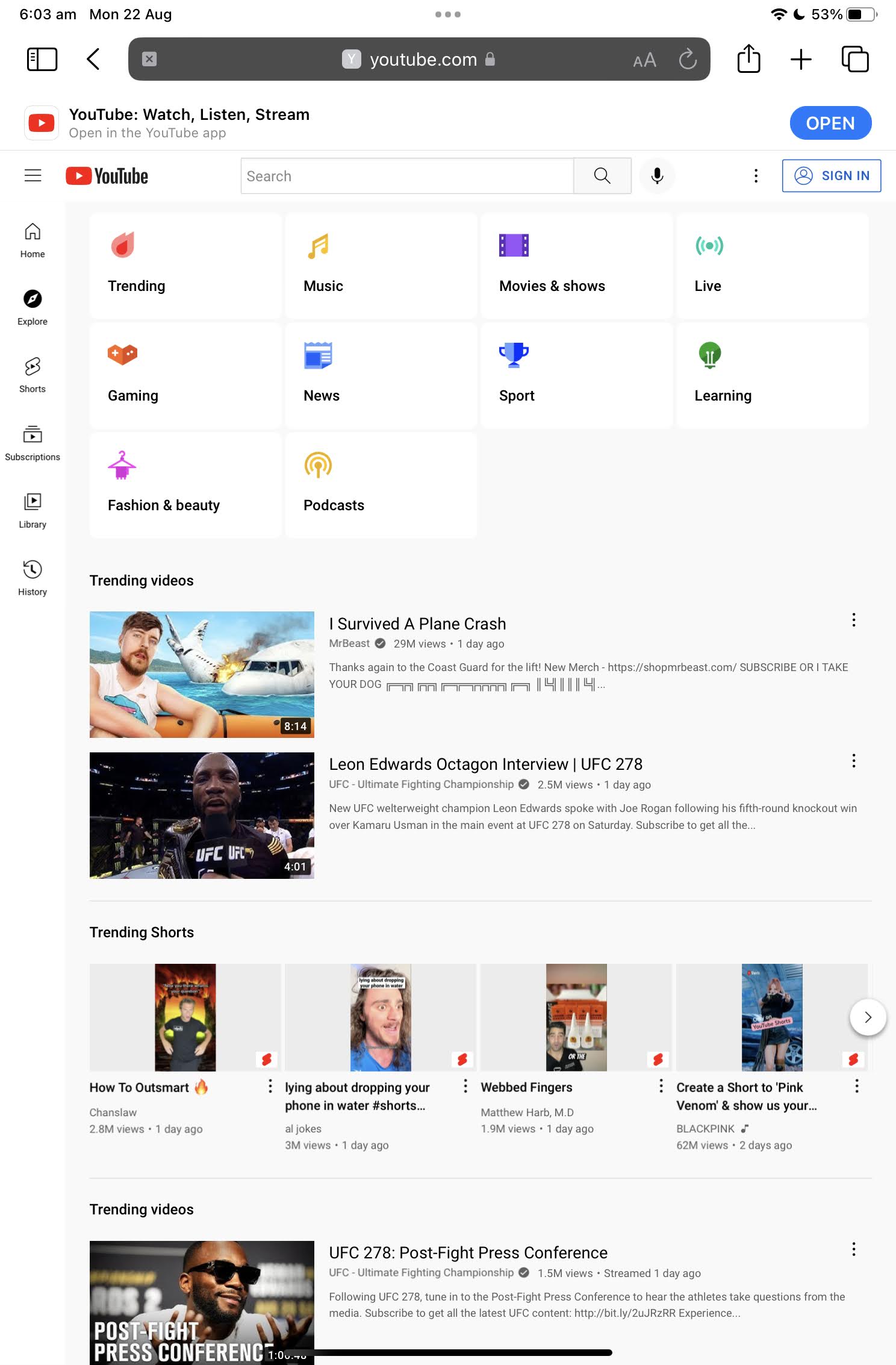This photo captures a screenshot of the YouTube homepage, likely taken from a cell phone. At the top of the screen, cell phone status icons are visible on both the right and left sides. Below these icons, the URL "youtube.com" is displayed inside a gray navigation bar. Underneath the navigation bar, there is a banner that reads "YouTube: Watch, Listen, Dream" with an option to open the YouTube app.

Further down, the interface shows a YouTube logo and a search bar. Below the search bar, various category icons are aligned horizontally, functioning as buttons for quick access to sections such as Trending, Music, Movies & Shows, Live, Gaming, News, Sports, Learning, Fashion & Beauty, and Podcasts.

At the bottom of the screenshot, the "Trending Videos" section is prominently displayed. The first video features Mr. Beast with the title "I Survived a Plane Crash." The second video, taken from UFC 278, features Leon Edwards' octagon interview and has garnered 2.5 million views.